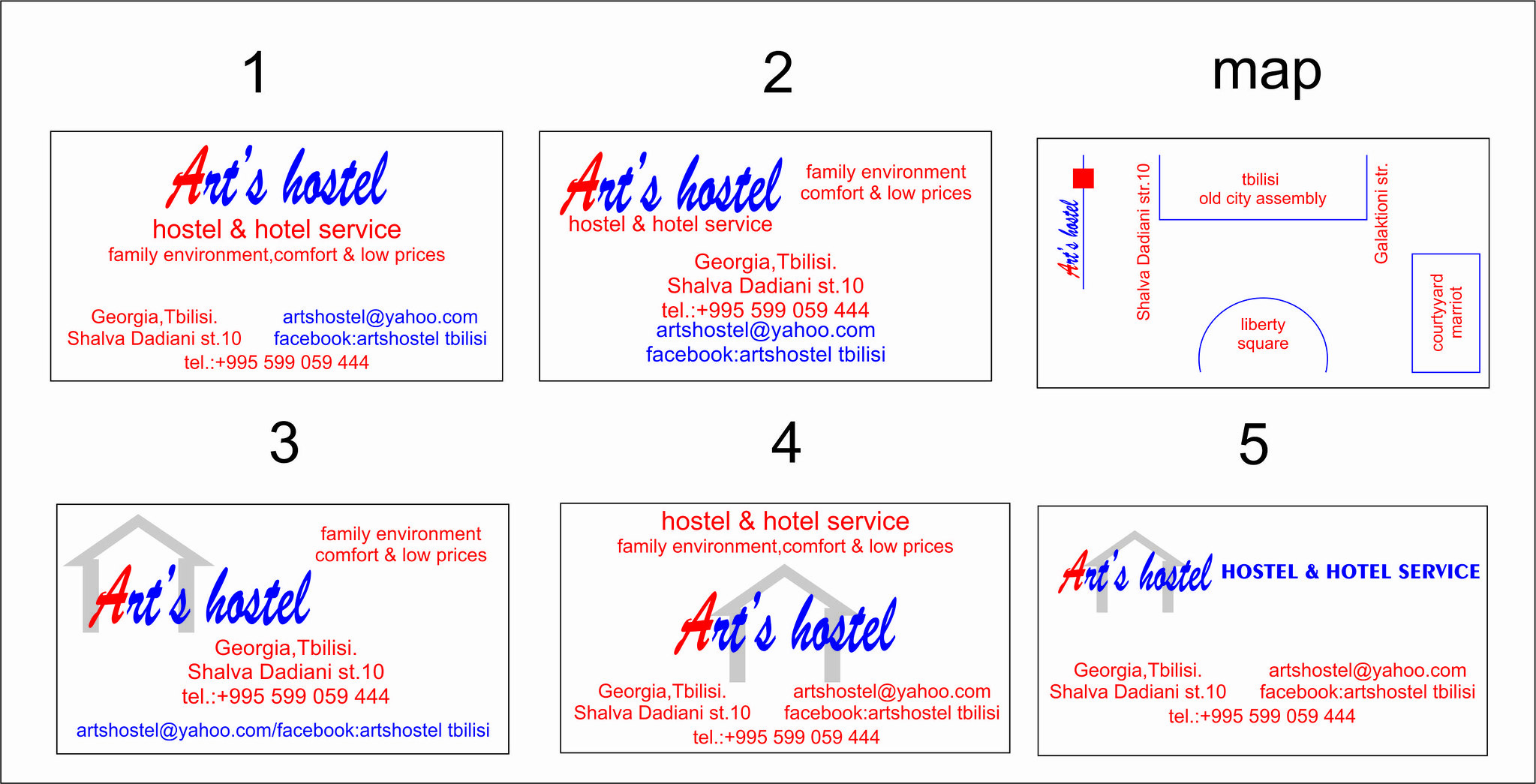This image displays five variations of a business card for "Arts Hostel," each emphasizing a family environment, comfort, and low prices. All cards feature blue and red text on a white background, with the prominent "A" in "Arts" colored red. The consistent elements across all variations include:

- Title: "Arts Hostel"
- Subtitle: "Hostel and Hotel Service"
- Slogan: "Family Environment, Comfort, and Low Prices"
- Location: Georgia, Tbilisi, Shalva Dadiani Street 10
- Contact: Email (artshostel@yahoo.com), Facebook (Arts Hostel), and a telephone number (+995-599-059-444).

Three of the cards incorporate a grey house logo, enhancing the homely feel. Some variations include a small map, marked with key landmarks such as "Tbilisi Old City Assembly" at the top center, "Liberty Square" at the bottom, "Courtyard Marriott" to the right, "Shalva Dadiani Street 10" to the left, and "Galaktiani Street" to the right of the assembly.

Design details vary, with text arrangements and logo placements differing slightly, offering diverse layouts while maintaining the core information and aesthetic consistency.